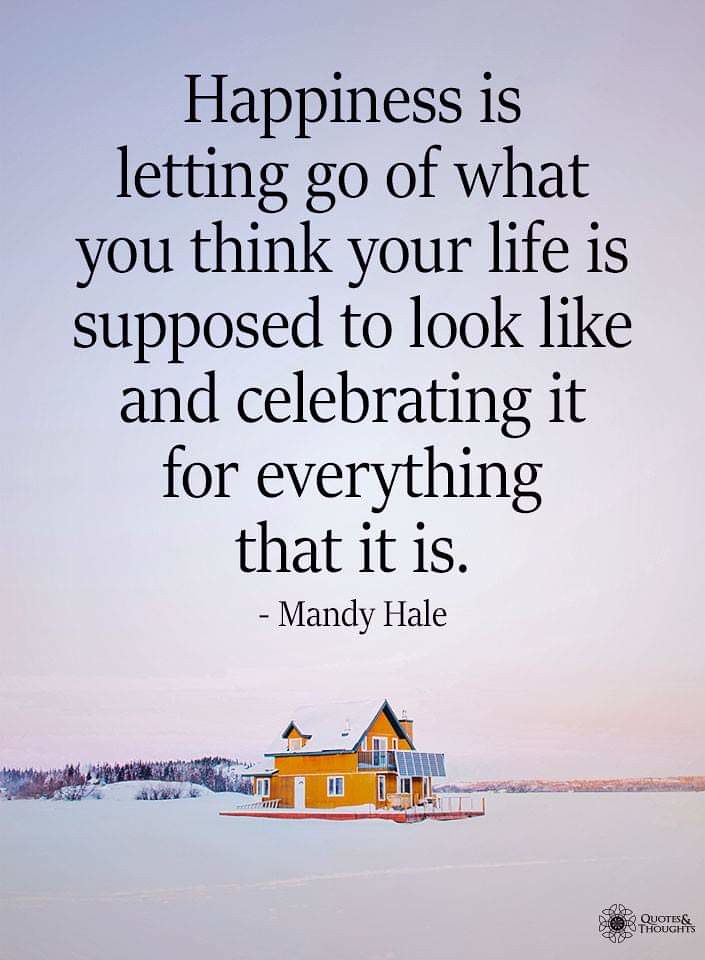This tall rectangular photograph, reminiscent of a greeting card, features an inspirational quote at the top in bold black font: "Happiness is letting go of what you think your life is supposed to look like and celebrating it for everything that it is," attributed to Mandy Hale. Below the quote, in the bottom right corner, a smaller text reads "quotes and thoughts" alongside a small illustration of a flower. 

The image backdrop presents a serene and snowy rural scene. At the picture's lower quarter, there is a several-story, gold-colored wooden house with snow blanketing its roof. The house is set atop what appears to be a red structure and features both a front porch with an A-frame awning and a back porch. This picturesque house sits within a flat, expansive white snowfield. To the left, black and purple-hued trees, also covered in snow, hint at a dense forest, while a thinner horizon line is visible to the right. Above this tranquil scene, the sky transitions from a warm pink near the horizon to a light blue at the top of the photograph.